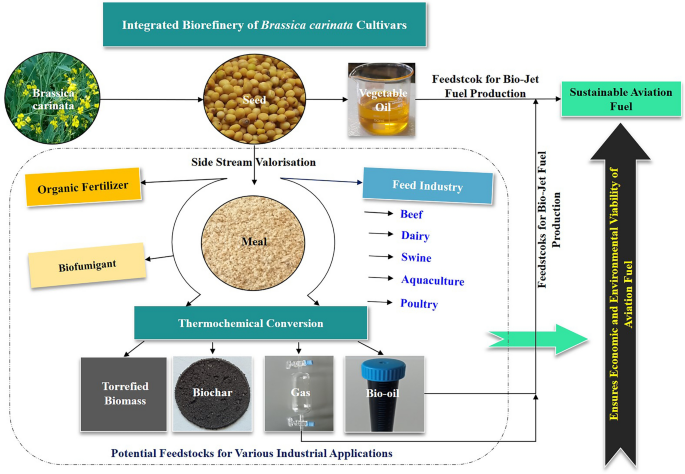The infographic diagram titled "Integrated Biorefinery of Brassica carinata Cultivars" appears in a turquoise rectangle at the top, suggesting it could be used in an educational setting like a textbook or college classroom. The diagram illustrates the process of producing sustainable aviation fuel from Brassica carinata plants through multiple pathways. 

At the beginning of the process, a circular photo of Brassica carinata plants leads to another circle containing an image of seeds labeled "Seed." From the seed, two main pathways are depicted. One pathway shows an arrow leading to vegetable oil production, followed by another arrow labeled "Feedstock for biojet fuel production" which ultimately points to a green box labeled "Sustainable Aviation Fuel."

The second pathway from the seed leads downward to a complex diagram labeled "Sidestream Valorization." It starts with the seed converting to "Meal," from which various arrows branch out, leading to "Organic fertilizer," "Biofumigant," feed industries for "Beef, dairy, swine, aquaculture, and poultry," and "Thermochemical conversion" producing "Torrefied biomass, biochar, gas, and bio oil." This section is labeled "Potential feedstocks for various industrial applications," with another arrow pointing to "Feedstocks for biojet fuel production" that eventually converge into the same "Sustainable Aviation Fuel" box.

To the far right of the diagram, a prominent black arrow emphasizes that this biorefinery process "Ensures economic and environmental viability of aviation fuel." The detailed interconnections and specific terminologies highlight the comprehensive approach to creating sustainable fuel and various by-products from Brassica carinata.